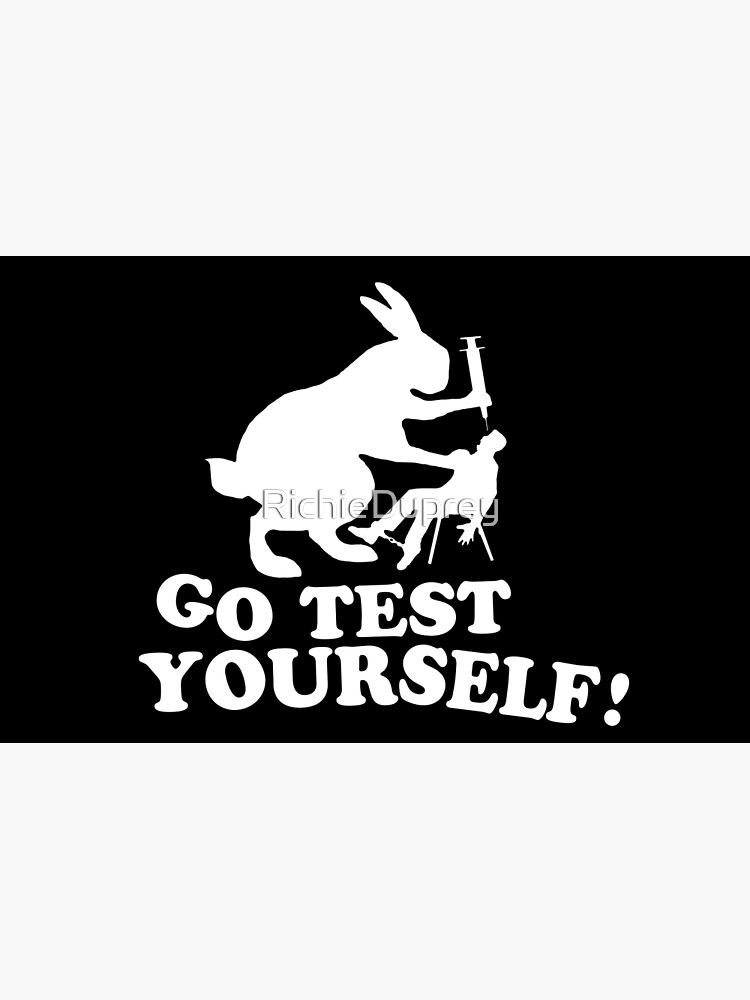The image is a stark black and white illustration evocative of an animal rights protest sign or t-shirt. Central to the image is a large white silhouette of a menacing rabbit wielding a giant syringe, poised to inject a terrified man who sits shackled by his ankles to a chair. The man's silhouette, also white, shows him recoiling in fear, mouth agape and arms restrained behind the chair, a grim depiction likely symbolizing the horrors of animal testing. Above the scene, bold white text commands, "Go Test Yourself!" emphasizing the anti-animal testing message. Additionally, a semi-transparent watermark reading "Richie Dupre" identifies the artist responsible for this poignant graphic.